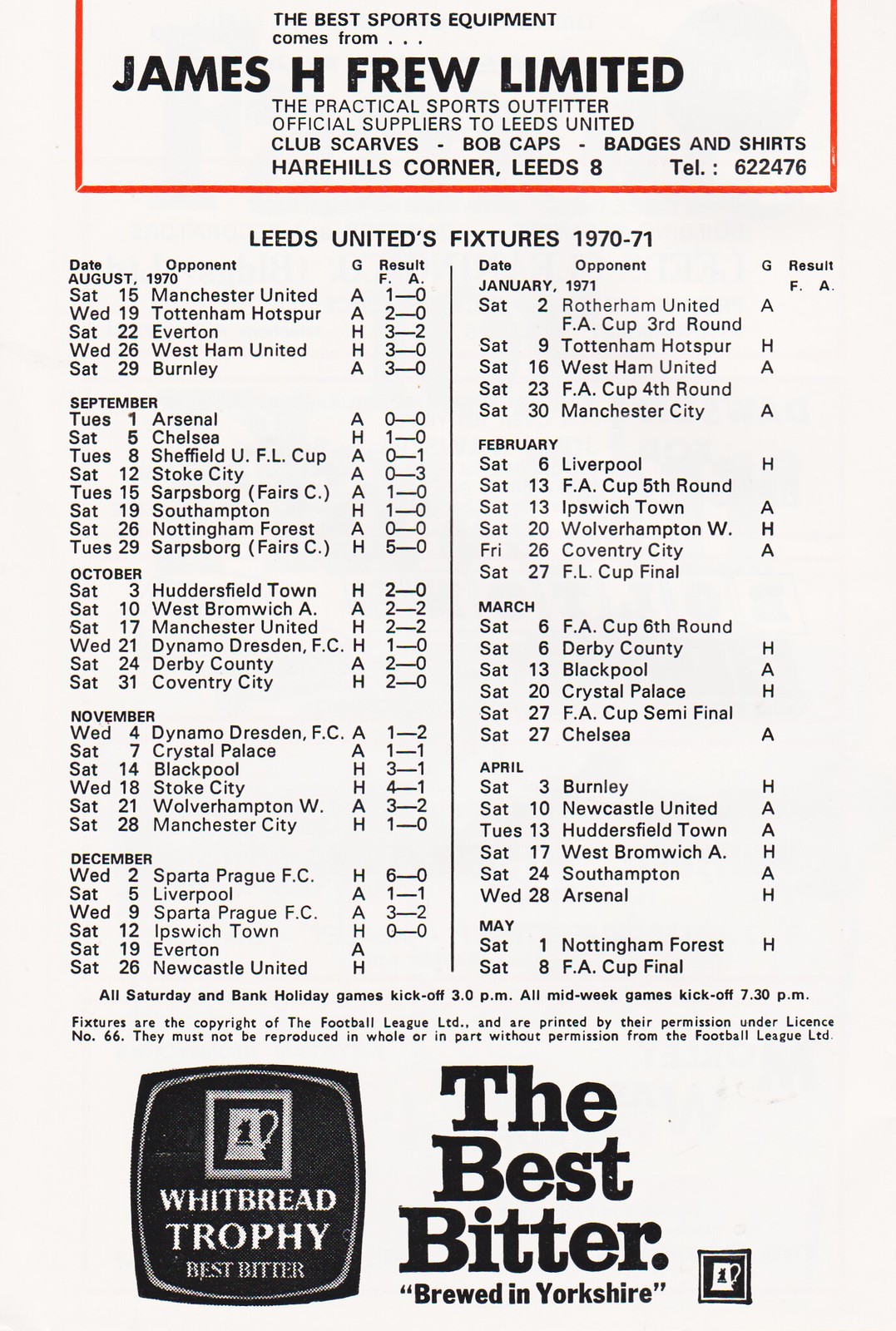This image features a detailed page from a sports program, showcasing a game schedule for Leeds United's fixtures for the 1970-71 season. The background is predominantly white, adorned with a narrow red frame along the top edge. Within this red frame, an advertisement is prominently displayed, stating, "The best sports equipment comes from James H. Frew Limited, the practical sports outfitter, official suppliers to Leeds United, club scarves, bobcaps, badges, and shirts." Also included is the company's contact information: Hare Hills Corner, Leeds 8, telephone 622-476.

Beneath the advertisement, the schedule for Leeds United's fixtures for the 1970-71 season is meticulously laid out. The chart lists the dates, opponents, game locations (home or away), and results of the matches. It begins in August 1970 with a match against Manchester United on Saturday, August 15th, which Leeds United won 1-0. The schedule continues through to May 1971, with entries for each month displayed on the left-hand side for the latter half of 1970 and on the right-hand side for the first half of 1971. Scores have been filled in up to December 12th, 1970.

At the bottom of the page, there is an advertisement featuring the logo for Whitbread Trophy Best Bitter, accompanied by the text, "The Best Bidder, brewed in Yorkshire." This thorough depiction captures both the excitement of the sporting fixtures and the prominence of James H. Frew Limited as a key supplier of sports equipment.